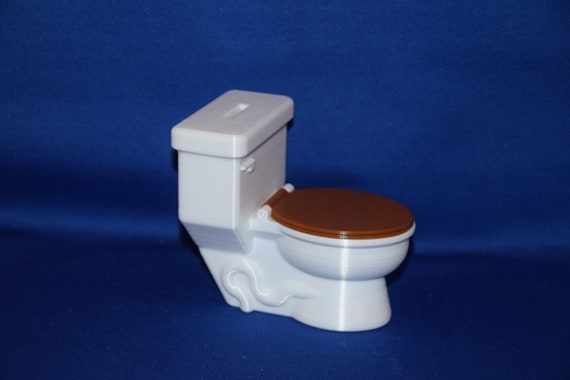The image is a detailed color photograph, captured in landscape orientation, featuring a small, modeled toilet that appears to be made of clay or a similar material. The toilet is oriented sideways with the tank on the left side of the image and the bowl on the right. It is primarily white, mimicking porcelain, with a shiny surface, though it is uncertain if it is actually porcelain. The most striking feature is the dark wooden brown lid, which is closed, along with a matching brown seat. The toilet includes various raised details, such as a non-functional flush handle and the plumbing line at the base. Notably, the tank has a slit on its top, suggesting that this model could serve as a piggy bank. The background is a royal blue, resembling folded fabric, covering both the back wall and the floor, creating a stage-like appearance for the toilet model. The style of the photograph is representationalism realism, emphasizing the miniature toilet's conventional design and realistic features.